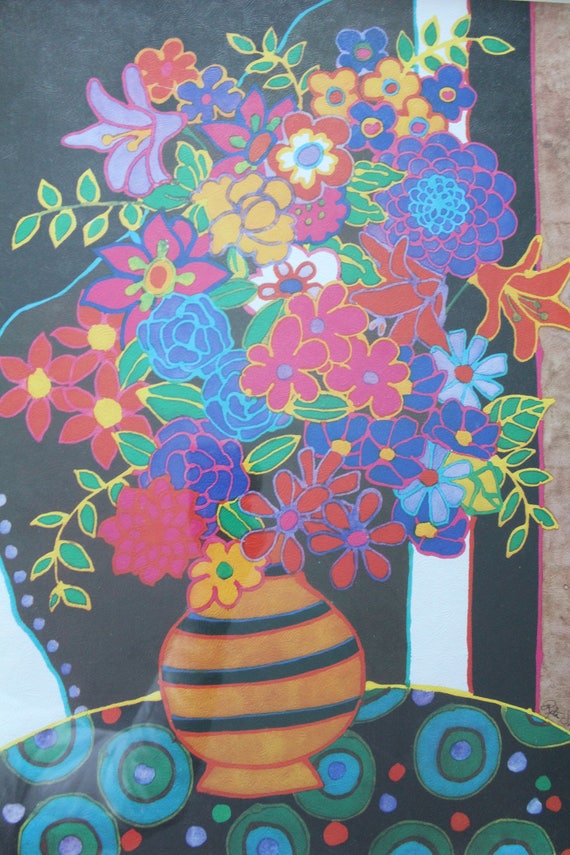This vibrant color image portrays a detailed scene, likely a photo or a depiction of art. The photograph seems to capture a piece of art installed on a surface with reflective properties and noticeable color variations, suggesting it could be a wall covering or a rug. The artwork showcases a beautifully intricate table with a mosaic design. This round table features a black background adorned with large concentric circles in shades of blue and green, creating an eye-catching pattern. Atop the table sits an ornate vase, boldly colored in gold and black stripes reminiscent of a bumblebee. The vase is overflowing with an exuberant bouquet of flowers in vivid hues of oranges, reds, yellows, and greens, which dominate the upper portion of the image. The background contains sections of black and white, making the colorful elements of the vase and flowers pop dramatically, evoking a sense of brilliance and liveliness.